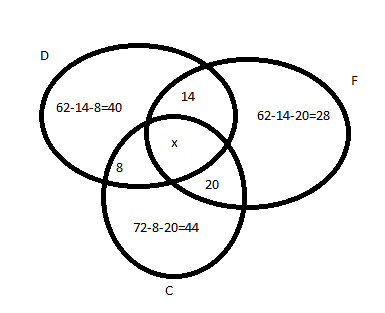This is a detailed drawing featuring three interlinked circles, each marked with distinct letters and numbers. 

In the upper left, there is a black circle labeled "D." Within this circle, the equation "62 - 14 - 8 = 40" is prominently displayed. Towards the lower part of this circle, you will find the numbers "8," "X," and "14."

On the right side of the drawing, another black circle is labeled with the letter "F." Inside this circle, the equation "62 - 14 - 20 = 28" is featured. At the lower part of this circle, the number "20" can be seen.

The third and smallest circle is marked with the letter "C." Within this circle, the equation "72 - 8 - 20 = 44" is visible. 

All three circles intersect at various points, with the numbers "8," "X," "20," and "14" interlocking with each circle, creating a cohesive and intricate pattern.